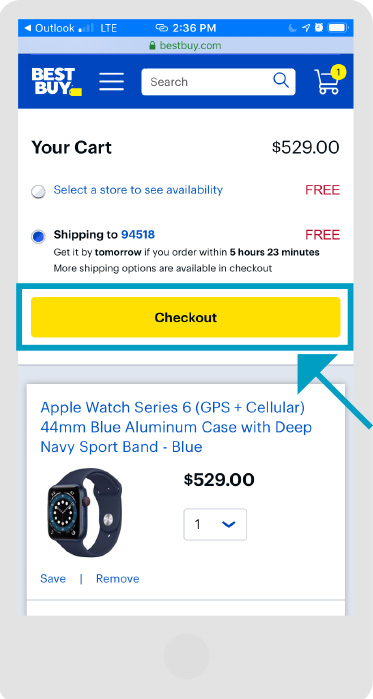A screenshot of the Best Buy website interface displays various elements against a gray background. In the top left corner, the recognizable yellow Best Buy tag logo is present, next to a shopping cart icon featuring a yellow circle with the number "1" in black text. 

A search bar, with a hamburger menu icon to its left and a magnifying glass inside, is prominently positioned at the top. To the right of this bar, the background is blue. The website depicted is "bestbuy.com," and at the very top, there is a time display reading "2:36 pm" within an alarm clock symbol.

Further details include the user's shopping cart total of "$529" and a blue radio dial button indicating "Select a store to see availability." Below this, the text "FREE SHIPPING to 94518" is shown in red, and another blue-shaded radio dial emphasizes the free shipping offer. Highlighted in bold text is the message "Get it by tomorrow if you order within 5 hours 23 minutes," followed by a note that "More shipping options are available at checkout."

Towards the bottom of the interface, a prominent yellow rectangle with a blue border contains the word "CHECKOUT" in black text. An accompanying blue arrow points to this yellow rectangle, drawing attention to the checkout option.

The product featured is an "Apple Watch" described in blue text as "Apple Watch Series 6 (GPS + Cellular, 44mm) Blue Aluminum Case with Deep Navy Sport Band."